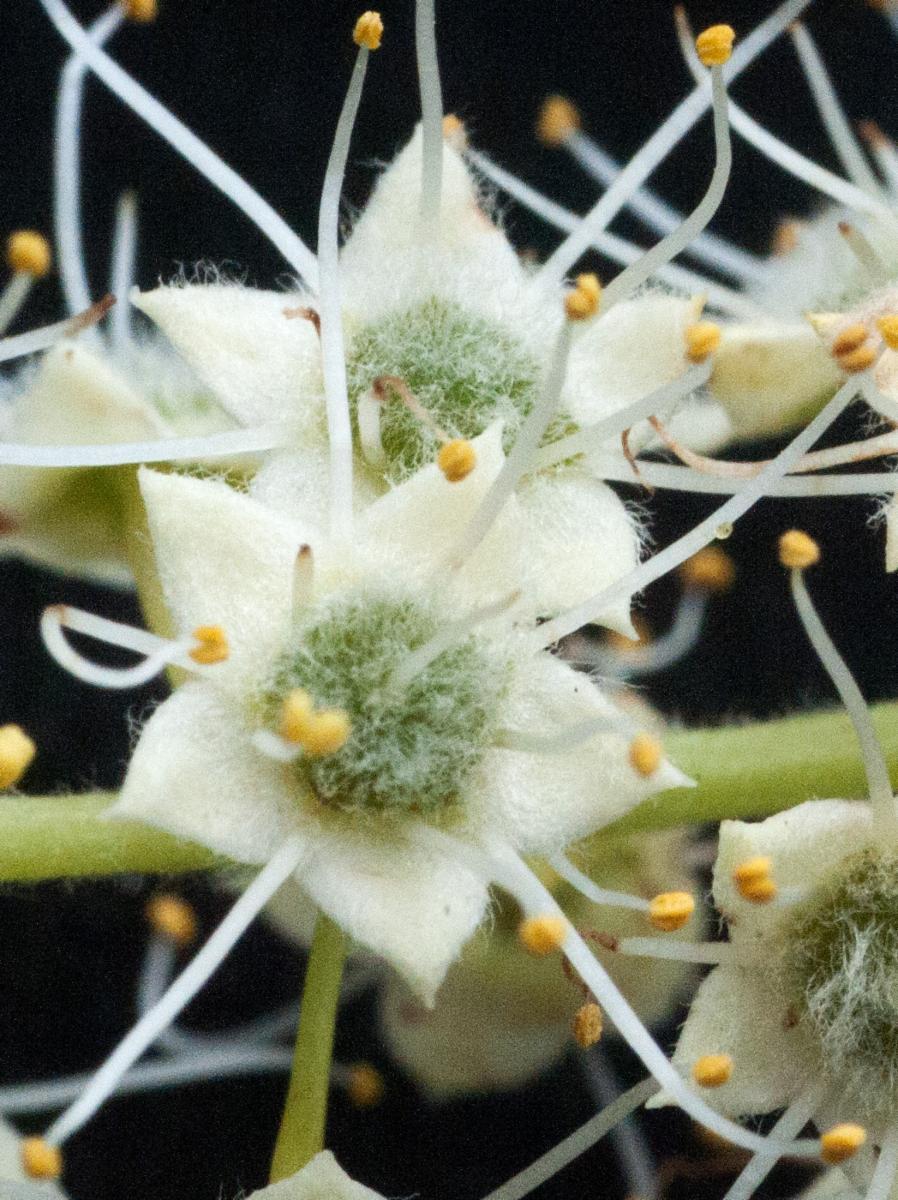This image displays a close-up of several small, white flowers with triangular petals, each adorned with fuzzy textures. The flowers' centers are green, from which numerous fuzzy, white tentacle-like structures, tipped in yellow, extend outward. The fuzziness of the flowers almost gives them the appearance of being crafted from felt, lending them an unreal, movie-like quality. Set against a solid black background, the flowers' white tones and textural details are highlighted distinctly, enhancing their vibrant and unique appearance.